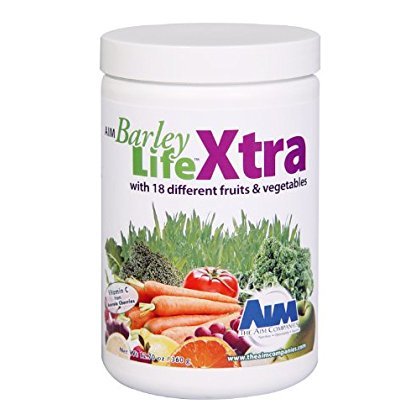This product image showcases a white, cylindrical plastic canister with a white screw-on lid, labeled "Barley Life Extra" by The AIM Companies. The label, set against a pure white background, prominently features the product name with "Barley" in green, "Life" in a larger green font, and "XTRA" in purple. Below this, black text states "With 18 different fruits and vegetables." The label includes a vibrant collage of various fruits and vegetables such as wheatgrass, kale, tomato, carrots, cherries, lime, lemon, orange, grapes, green apple, broccoli, and a strawberry. A small label on the left highlights "Vitamin C," and the company’s logo, "AIM," is displayed on the right along with their web address, www.theaimcompanies.com. The net weight of the product is 360 grams, indicated at the lower left corner.